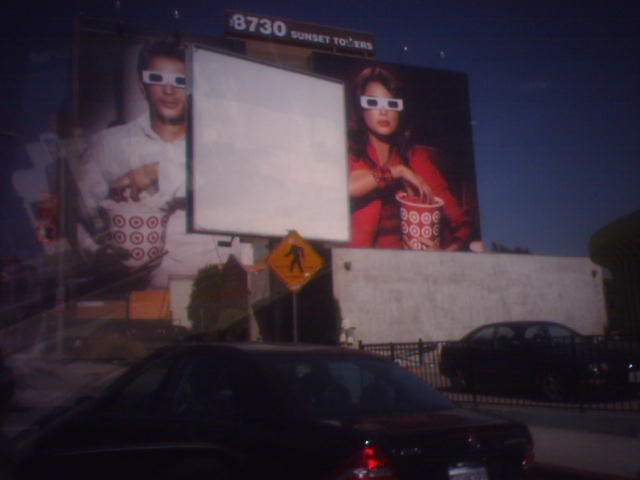A nighttime outdoor scene captures a large wall with a projected image featuring a man and a woman both wearing 3D glasses. The man on the left is seen dipping his hand into a white bucket adorned with red target symbols, resembling a popcorn container. The woman on the right, dressed in a red blouse, reaches into a red bucket with white target symbols, seemingly filled with red food. Above the projection, partially obscured text reads "8730 Sunset to...". In the foreground, a yellow diamond-shaped street sign with a black border and the symbol of a person walking indicates a pedestrian crossing. At the base of the display, two cars are visible: one parked in clear view and another partially obscured behind a black metal fence. The image appears somewhat grainy and blurry due to the low light conditions of the night.